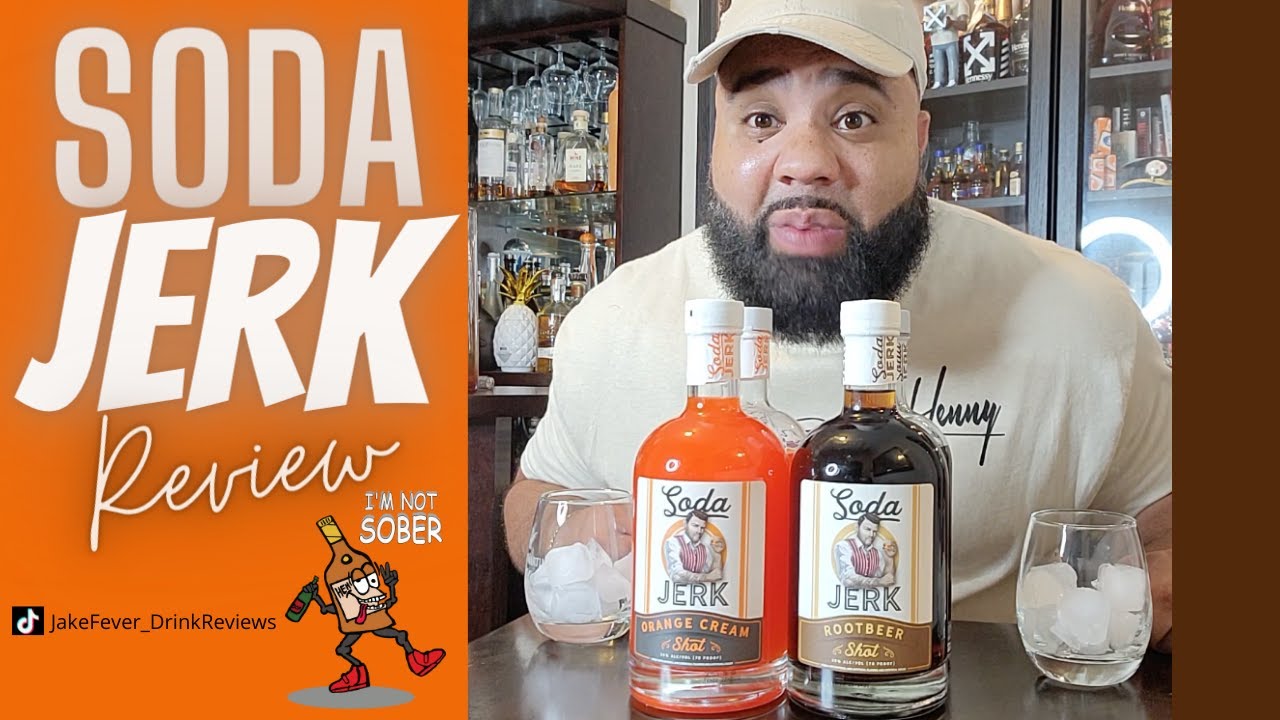In this detailed advertisement for the Soda Jerk Review, a black man with a neatly trimmed beard and a beige hat gazes into the camera with a curious, smirking expression. He wears a light-colored shirt inscribed with "Henny" or "Henry" in cursive, adding a casual touch to his appearance. The setting appears to be a bar adorned with various indistinguishable bottles and glasses in the background. In the foreground, bottles of Soda Jerk flavored beverages take center stage: an orange bottle labeled Soda Jerk Orange Cream and a brown one labeled Soda Jerk Root Beer. Flanking these bottles are two glasses filled with ice, ready for tasting. To the left of the image, a vibrant orange background prominently features the bold text "Soda Jerk Review" alongside a whimsical cartoon of a tipsy anthropomorphized bottle holding another bottle, with the words "I'm not sober" playfully integrated. Below the cartoon is the social media handle "JakeFever_DrinkReviews," hinting at the content's origin likely linked to TikTok or YouTube.